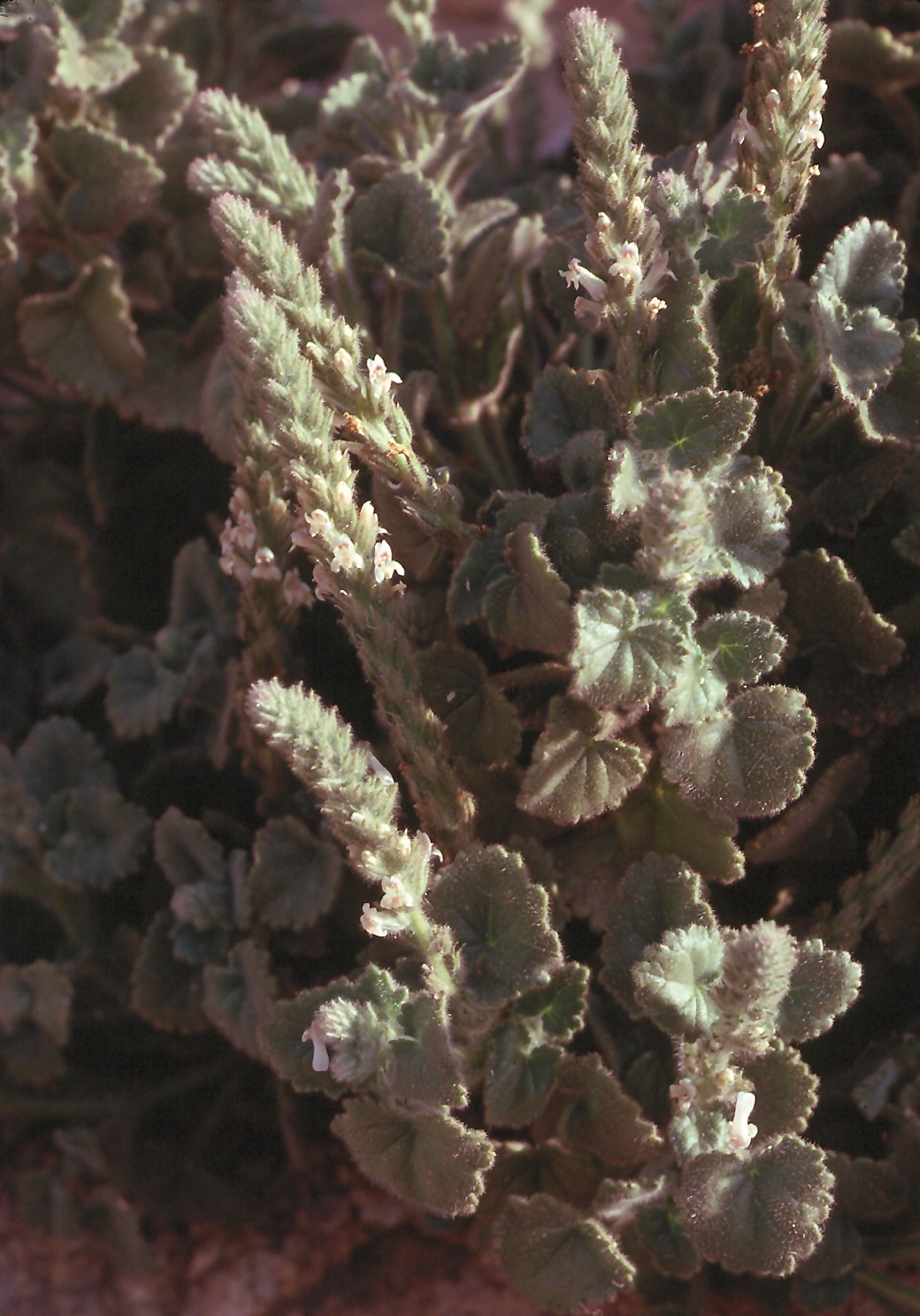Aerial portrait view of a desert-like garden, dominated by a variety of small, medium-green succulent plants. The majority of the image showcases two types of vegetation: some with thick, meaty leaves, possibly cactus-like, and others with thin, tall flowery stalks resembling wheat. The sunlight forms distinct lines, illuminating about the top 20% and creating sporadic highlights at approximately 20% and 60% from the left. The base of the image reveals a touch of brownish-tan brush, while sporadic touches of light green and pink colors add contrast. These plants are randomly scattered across the frame, giving a wild, natural aesthetic with no visible text, indicating it might have been taken in a garden or outdoor setting.